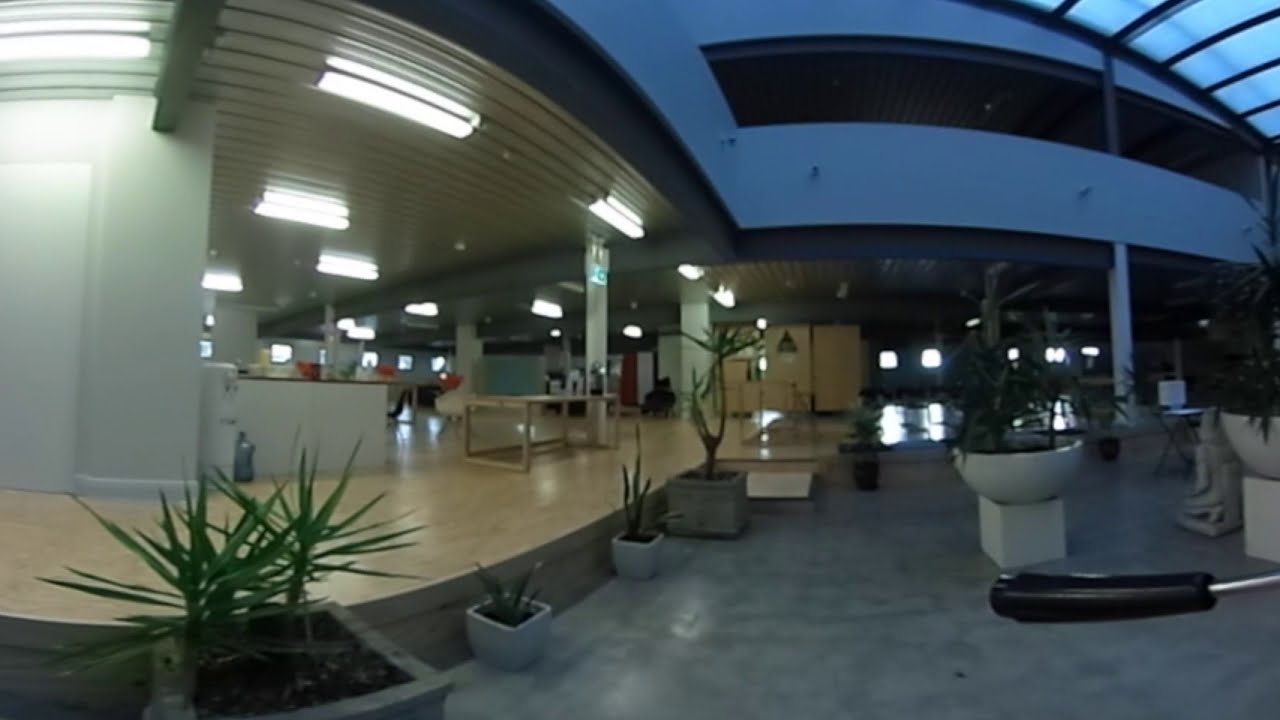The image depicts an interior of a semi-outdoor commercial space, possibly a shopping center or hotel lobby, illuminated by natural light from a skylight visible at the top right corner. The setting features a variety of flooring types, including shiny tile on the right side and hardwood on the left. A handlebar, potentially from a shopping cart or vehicle, is partially visible in the foreground. The space abounds with greenery, including decorative plants on both sides and towards the center, positioned in white containers.

On the left, the space includes a white-walled area with tables, chairs, and a bar or serving area beneath ceiling lights. This zone steps up into a slightly elevated section characterized by brown tile flooring. There's a gathering of people around what seems to be a lobby or desk area, partially obscured by a couple of pillars.

The ceiling features a glass or see-through atrium with structural bars, letting in ample daylight. The color palette of the image is diverse, including shades of gray, white, brown, green, light blue, tan, orange, and red, providing a harmonious yet vibrant atmosphere.